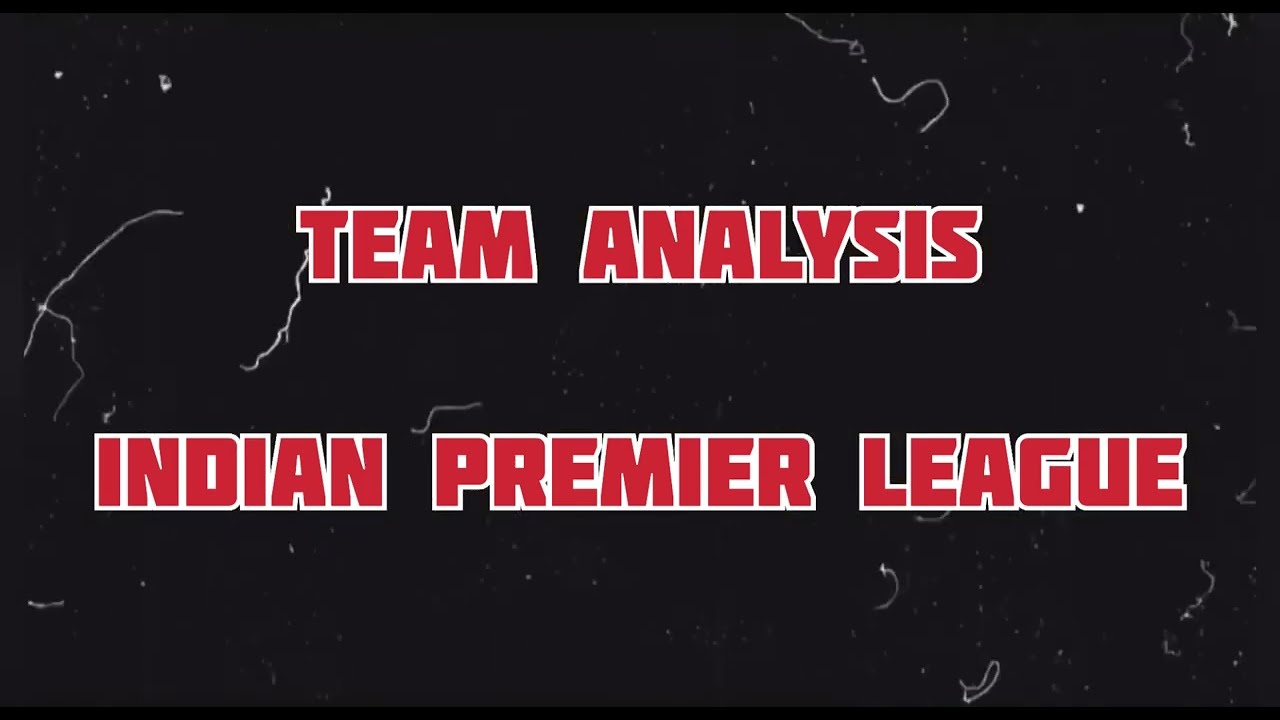The image is a monochrome design with a title prominently displayed in the center. The background is black, deliberately styled to mimic the appearance of aged film, complete with white squiggly lines and specks that resemble scratches and dust. Over this vintage-themed backdrop, bold text appears in all uppercase letters. The top line, slightly above the midpoint, reads "TEAM ANALYSIS" in large red letters with white borders. Below this, in similarly styled red and white bordered letters, it reads "INDIAN PREMIER LEAGUE." The design suggests it could be a title screen for a video or a PowerPoint slide, possibly an introductory segment or title image for a visual presentation related to the Indian Premier League.